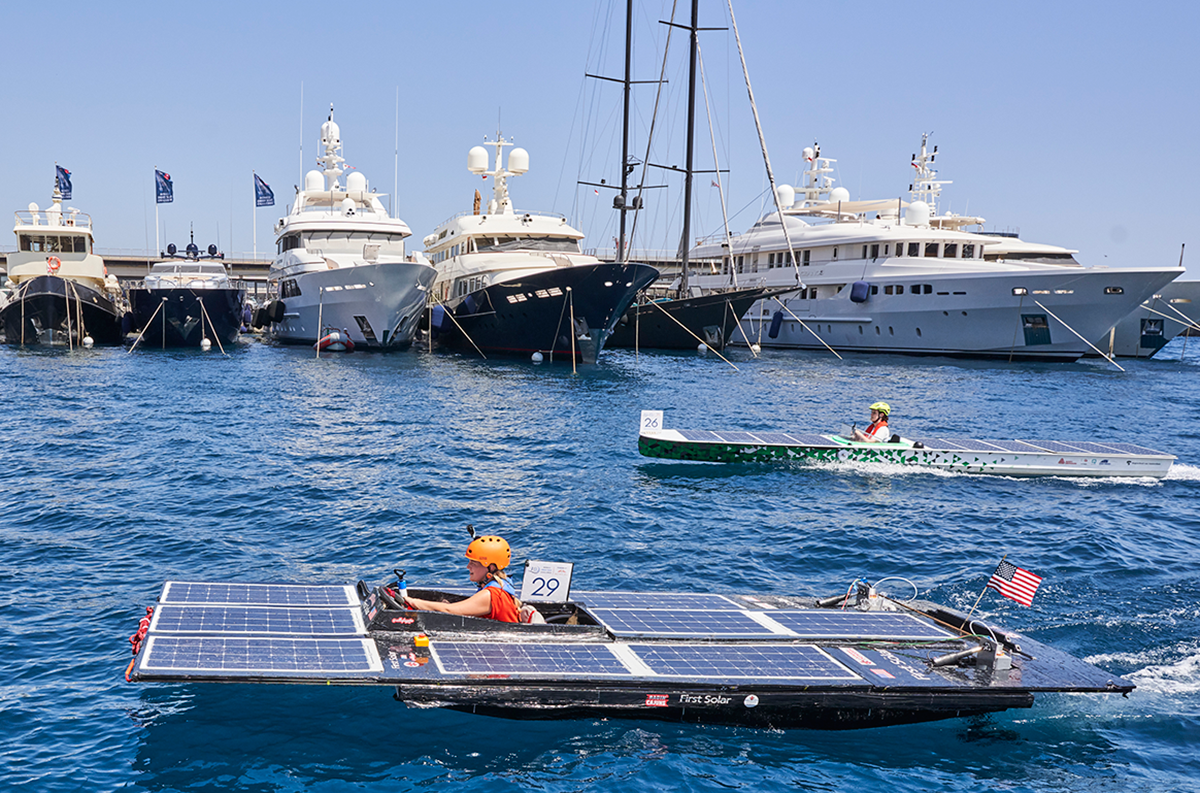The photograph showcases a vibrant scene of various boats floating on deep blue seawater. In the foreground, two sleek, flat boats equipped with solar panels capture the viewer's attention, each manned by a driver. The closest boat, marked with the number 29, features "First Solar" emblazoned on its side and an American flag at the stern. Its driver is identifiable by an orange helmet. Following closely behind is another boat, marked with number 26, piloted by a driver wearing a yellow helmet. Both boats appear poised for a race. In the background, a multitude of boats, including at least one large enough to be classified as a yacht, are anchored, their white and black hulls and towering masts creating an impressive maritime backdrop against the sky.